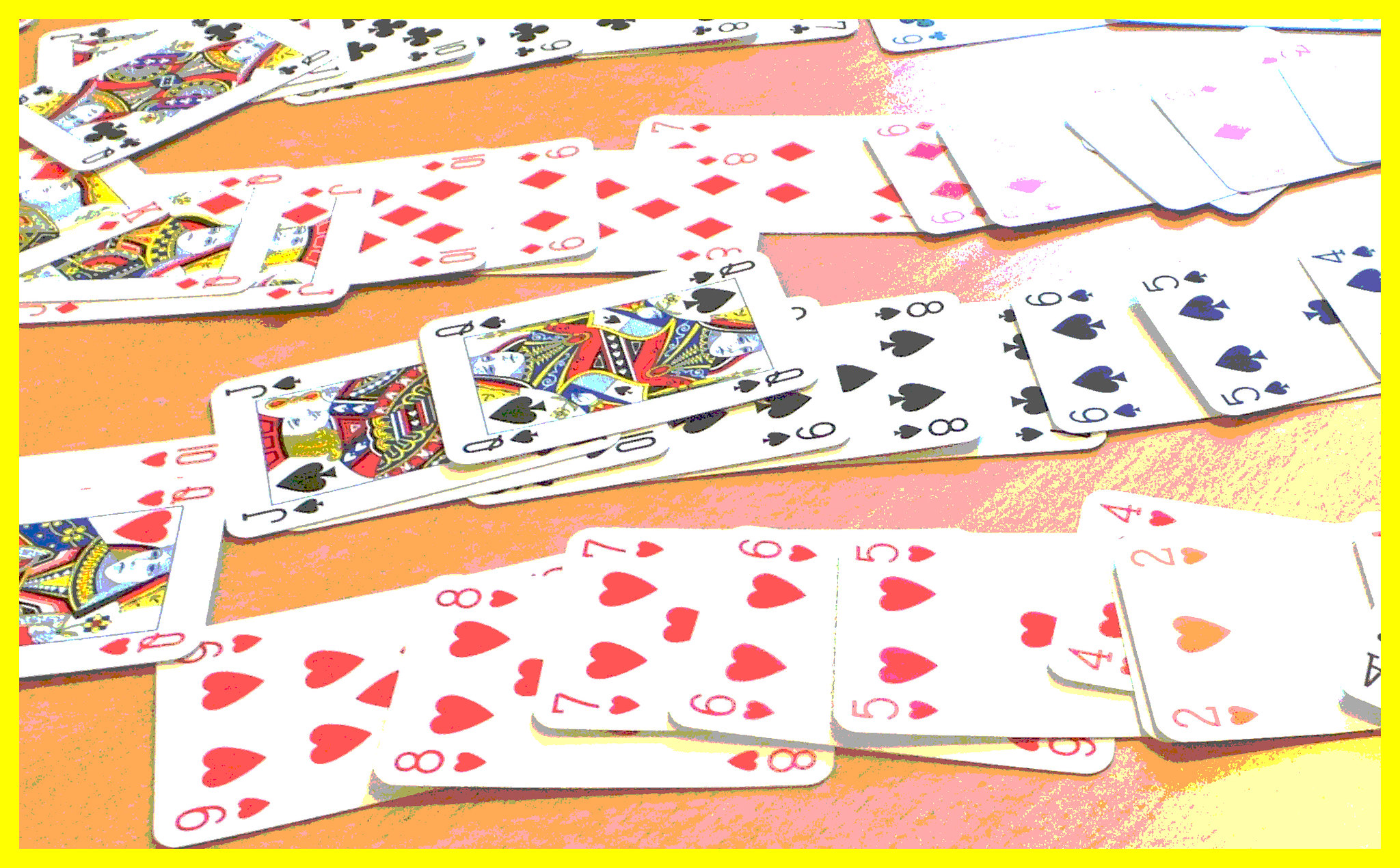An array of playing cards is meticulously laid out on a table, with each suit—hearts, spades, diamonds, and clubs—organized into individual columns. The cards are predominantly arranged in numerical order, although a few small discrepancies can be observed. Notably, the Queen of Clubs and the King of Diamonds are slightly overlapping each other. The image itself is rotated 90 degrees counter-clockwise, making the cards appear as if they are standing upright when viewed on its side. Despite the effort to organize, the alignment of the rows is somewhat imperfect, with cards overlapping in various places and not all rows perfectly straight. The table on which the cards are displayed reflects a nearby light source, adding a subtle gleam to the scene, suggesting someone might be preparing for a game like solitaire or simply arranging the cards for visual appeal.